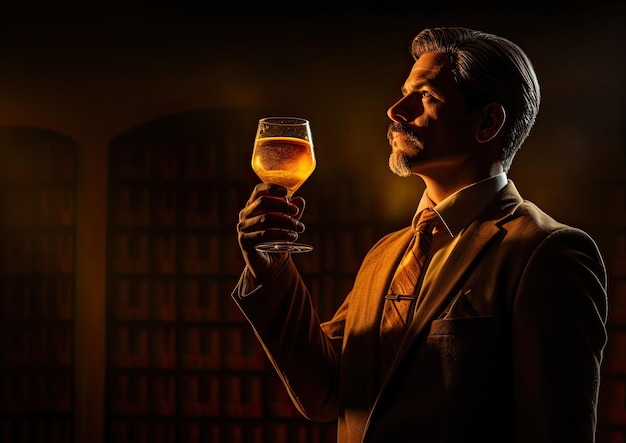The image portrays a distinguished man in a sharp brown suit with a coordinating tie and tie bar, exuding an aristocratic air. He sports a meticulously styled mustache and goatee, with hints of gray in his dark hair. The scene is bathed in warm, golden light, casting shadows that add depth to his contemplative expression as he gazes slightly upward, lost in thought. He holds a glass filled with beer, with light filtering through it, highlighting its amber hue. His other hand rests naturally, revealing his thumb, ring, middle, index, and pinky fingers. The background, gently out of focus, reveals a cozy, traditional setting with bookshelves and elegant woodwork, suggesting a library or formal room, enhancing the sophisticated atmosphere.